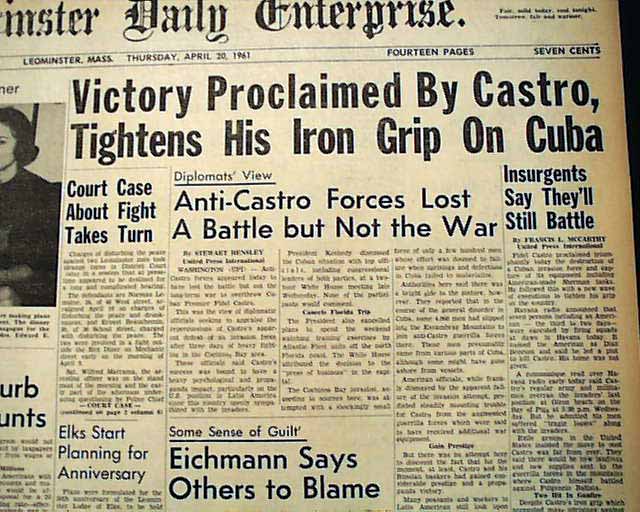The image depicts the front page of an old newspaper titled "Daily Enterprise" from Leominster, Massachusetts, dated Thursday, April 20, 1961. The newspaper consists of 14 pages and was priced at 7 cents. The paper has aged to an off-white, almost light beige color. The most prominent headline reads, "Victory Proclaimed by Castro Tightens His Iron Grip on Cuba." Below this, there's another bold article titled, "Anti-Castro Forces Lost the Battle but Not the War." Adjacent to these headlines, there is a partially visible black-and-white photograph of a woman on the left side of the page. Other articles on the front page include "Court Case About Fight Takes Turn," "Insurgents Say They'll Still Battle," "Elks Start Planning for Anniversary," and "Eichmann Says Others to Blame."